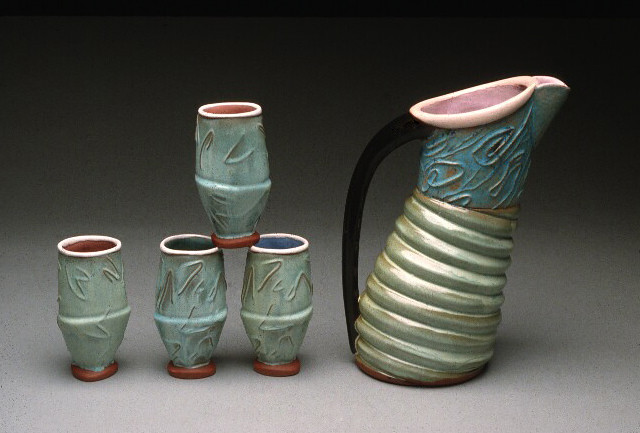This is a grainy photograph featuring a unique arrangement of ceramic pottery against a gradient background. The backdrop transitions from black at the top to a white-grey at the bottom, creating a striking visual effect. On the left side, four light blue-green cups, reminiscent of tall shot glasses or elongated egg cups, are arranged creatively. The leftmost cup stands alone, slightly set apart from the three others, with one of these three balanced delicately on the rims of the two beneath it. Each cup features intricate zigzag designs, a terracotta-colored rim at the base, and a white top with interiors varying between terracotta and blue.

On the right half of the image sits an elegant pitcher, designed to dispense liquid. This pitcher has a distinctive bird-like shape, with a long black handle extending from top to bottom. Its base is a ridged, shiny gold that occupies about two-thirds of its height. Above this, the pitcher transitions into a teal blue section, topped with a baby pink rim.

Overall, the contrasting hues and unique shapes make this a captivating composition of ceramic art.